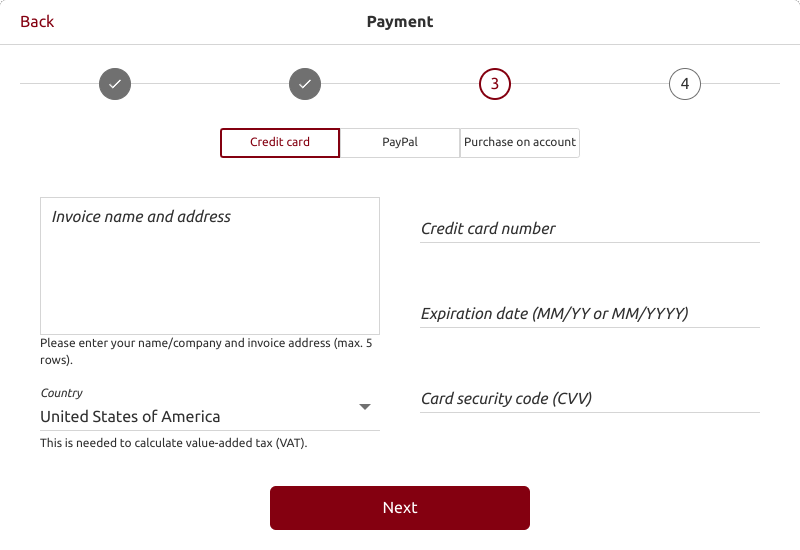The image displays a payment interface. At the top center, there's a bold black text that reads "Payment," while the top left corner features the word "Back" in red text. These elements are separated by a thin horizontal line running across the width of the interface.

Beneath this line, there is a progression bar with four icons. The first and second icons are circles with checkmarks inside them, indicating completed steps. The third icon is a red-bordered circle with the number "3" in red, signifying the current step. The fourth icon is a gray circle with the number "4" in gray, representing a future step.

Below the progress bar, there are three rectangular buttons. The first button, labeled "Credit Card" in red text, is followed by a "PayPal" button, and then a "Purchase on Account" button.

At the bottom left of the interface is a small boxed area labeled "Invoice Name and Address." To its right, three horizontal input fields are provided: the top field is labeled "Credit Card Number," the middle field reads "Expiration Date (MM/YY or MM/YYYY)," and the bottom field is labeled "Credit Card Security Code."